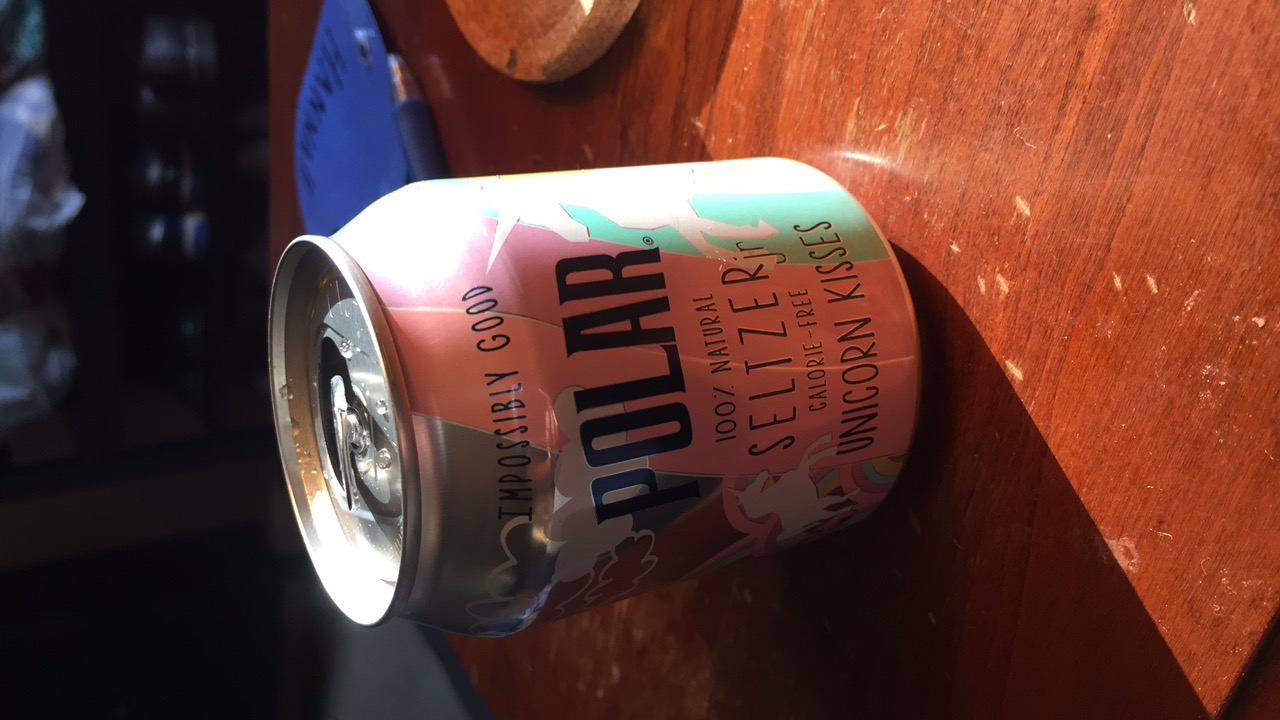This detailed caption consolidates and emphasizes the shared and repeated aspects of the descriptions:

This photograph captures a small, six-ounce can of Polar 100% Natural Seltzer labeled "Unicorn Kisses" sitting on a worn, medium-brown wooden coffee table with visible nicks and stains. The can is decorated with images of white unicorns set against backgrounds of pink, light purple, and light green colors, with additional design elements like stripes and possibly clouds or flowers blending throughout. The label prominently displays the words "Impossibly Good" at the top, although this text is somewhat difficult to read due to the light reflecting unevenly on the can. The can has been opened, with the traditional aluminum ring pull tab slightly up and residual droplets of liquid creating condensation marks around the mouth opening. Near the bottom, "Polar" is spelled out and accompanied by a copyright mark.